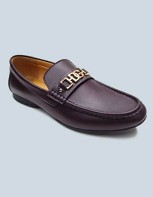This is a professional, close-up photograph of a high-end man's patent leather slip-on loafer. Crafted from deep brown leather, the shoe features meticulous hand-sewn seams and edges, contributing to its luxurious appearance. The interior is a rich tan color, complimenting the dark exterior. The shoe is adorned with an elegant, intricate brass embellishment that spans across the tongue. This design includes a series of geometric shapes, such as squares of varying sizes, fastened with gold balls. A small wooden heel adds a touch of sophistication. The shoe, positioned with the heel on the left and the toe on the right, stands alone against a backdrop of light blue, enhancing its striking features and ensuring it remains the focal point of the photograph.